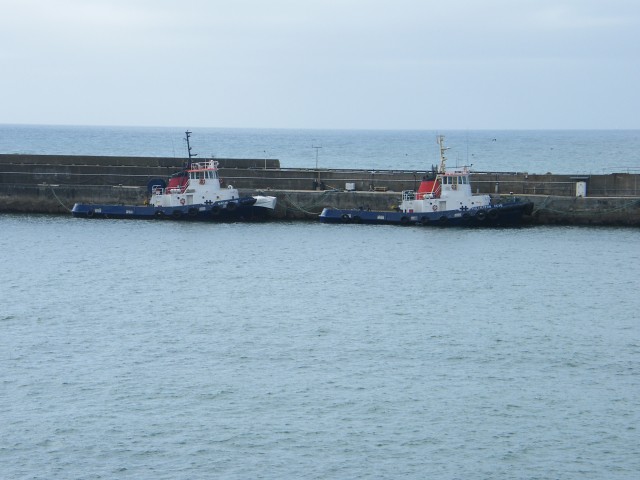This digital photograph captures an expansive, calm body of water, likely part of a large lake such as one of the Great Lakes or possibly an ocean, given the endless stretch of bluish-greenish-gray water merging with a pale, hazy blue sky on the horizon. Dominating the image is a massive barge that spans horizontally from one end of the frame to the other. The barge appears gray and forms a significant structure in the center of the picture. Flanking the barge are two nearly identical tugboats, crucial to maneuvering the large vessel. These tugboats feature black hulls and white wheelhouses. Their red exhaust funnels, capped with black, add a vivid contrast. The only distinguishing feature between the two tugboats is the color of the masts topped with electronic sensors and antennae: one is painted white, while the other is black. The scene is set under a light blue, cloud-streaked sky, adding to the tranquility of the image.